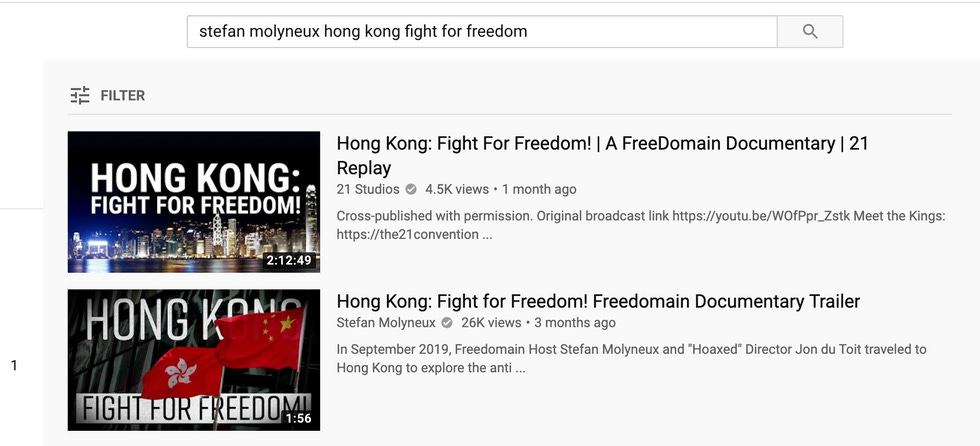This image depicts a website showcasing search results for "Stephen Milanuk's Hong Kong Fight for Freedom." In the search bar, the queried phrase appears prominently. Directly below the search bar, there is an option for filters accompanied by a clickable menu.

The primary visual focus is a photograph of Hong Kong, taken from across the water, with large white text overlaying the photo that reads, "Hong Kong Fight for Freedom." Adjacent to the photo in regular text, it says, "Hong Kong Fight for Freedom, a Free Domain Documentary, 21 replay. Cross-publish with permission. Original broadcast link," followed by a specific URL.

Beneath the main image is a secondary result showcasing two red Hong Kong flags, each adorned with a symbolic image. This section repeats the phrase, "Hong Kong Fight for Freedom, Free Domain Documentary Trailer." It further details that in September 2019, Free Domain host Stephen Milanuk and director John Dutroit traveled to Hong Kong to explore the situation. To read the full article, the viewer must click on the link, but currently, only these two search results are displayed.